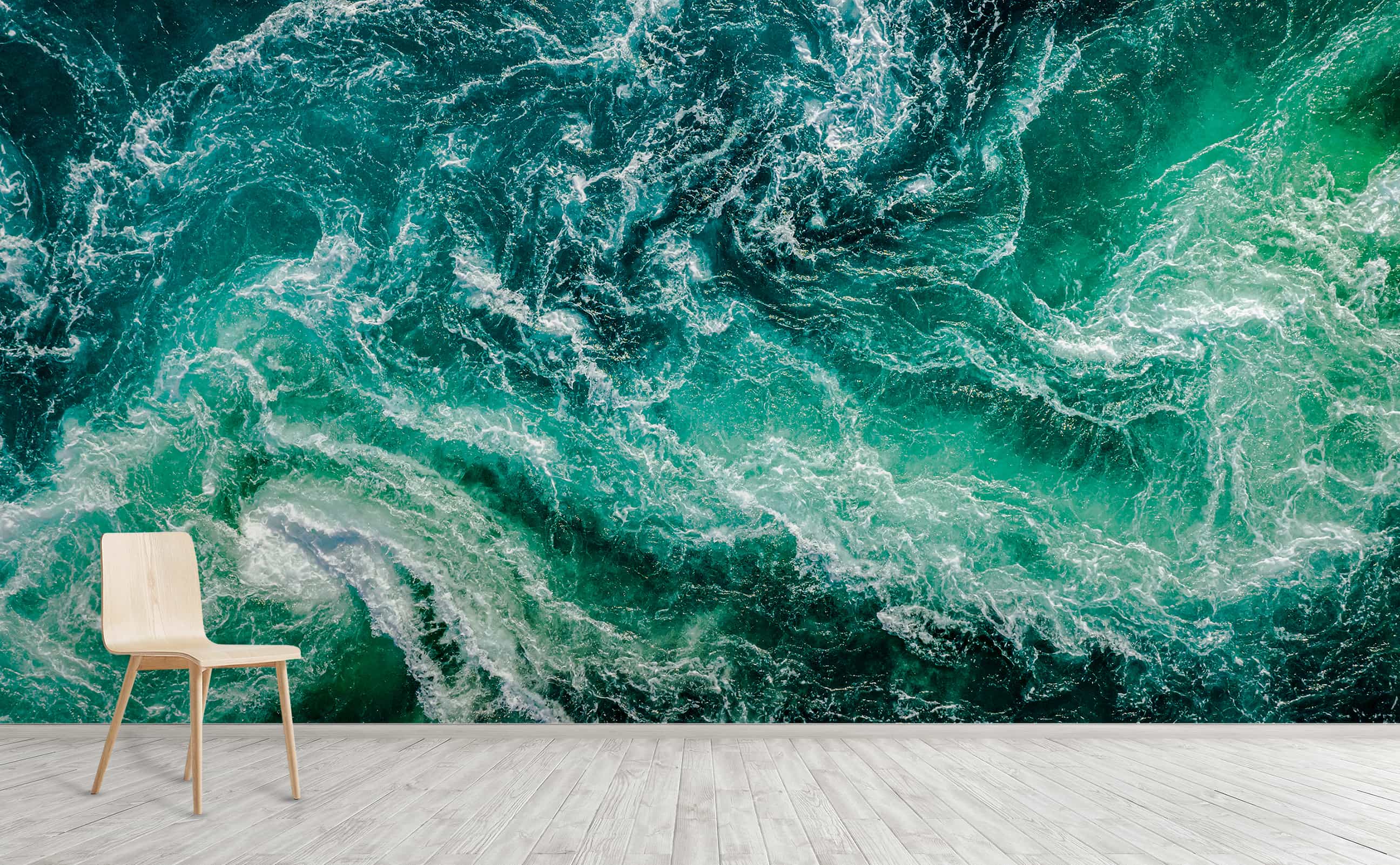The image showcases a minimalist room with a striking feature wall. The largest wall is adorned with a highly realistic design depicting an aerial view of a dynamic ocean scene, complete with swirling waves and white caps. The colors in the ocean range from dark green to lighter, almost lime green hues, interspersed with churning white foam. The intricate details make it unclear whether this artwork is a wallpaper, a large canvas, or perhaps a projection, but its vivid portrayal of the ocean's motion and depth dominates the space. The room's floor is a light grayish-beige wood or laminate, adding a subtle, neutral base to the scene. Positioned toward the left side is a simple, modern chair in a matching light beige color. The chair is skinny with a straight back and legs, devoid of any cushioning or decorative elements, emphasizing the room's clean and sparse aesthetic.